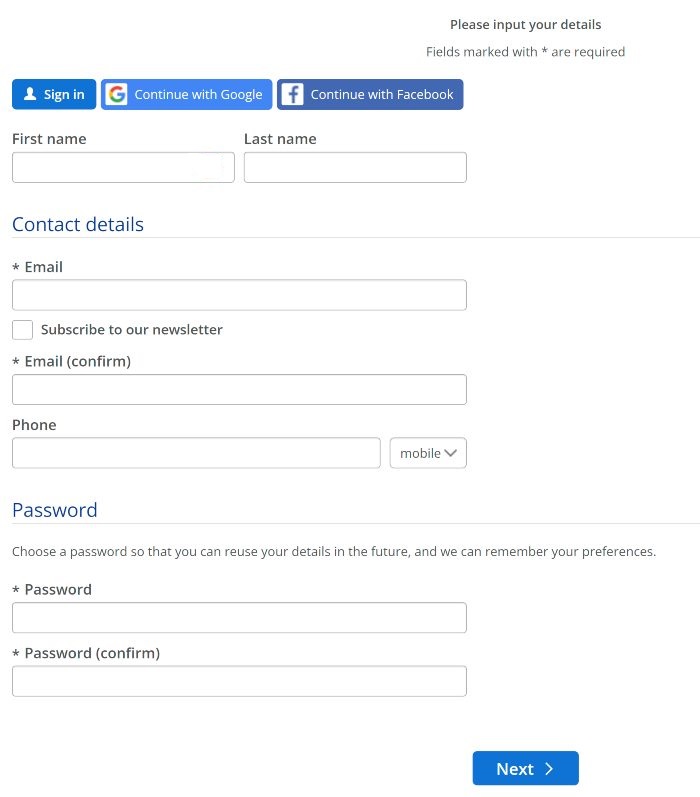The image features a user registration form set against a white background. The form header prompts users to "Please input your details," noting that fields marked with an asterisk (*) are required. Below the header are three blue buttons for account actions: 

1. A deep blue rectangle labeled "Sign In."
2. A lighter blue rectangle labeled "Continue with Google."
3. A deep blue rectangle labeled "Continue with Facebook."

The form includes several input fields:

- **First Name** (text box)
- **Last Name** (text box)

Under a blue section header labeled **Contact Details**, the form presents the following fields:

- **Email*** (text box with a star indicating it's required)
- **Confirm Email*** (text box with a star indicating it's required)
- **Phone** (text box)

Users can also opt-in to receive updates via a checkbox labeled **"Subscribe to our newsletter."**

In the subsection titled **Mobile and Password**:

- **Mobile** (text box)
- **Choose a Password*** 
  - Instruction: "Choose a password so that you can reuse your details in the future, and we can remember your preferences."
- **Confirm Password*** (text box)

Finally, at the bottom of the form, a prominent blue rectangle button labeled "Next" invites users to proceed to the next step.